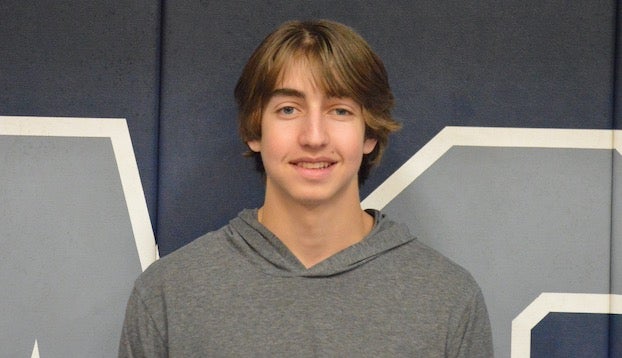This image features a close-up portrait of a young man, possibly a teenager, standing in front of a dark blue or black padded wall, which is likely found in a high school gymnasium. The wall padding appears to be divided into horizontal or vertical sections, designed to protect athletes. The padding displays light gray letters bordered in white, though their specific wording is not discernible due to the close-up nature of the photograph. The young man is dressed in a thin, gray, long-sleeve shirt with a hoodie, which lacks any visible logo or design. He has shaggy, curly brown hair extending down to his ears, thick eyebrows, and blue or hazel eyes, with one eye appearing slightly squinted. He also has a mole above his lip on the left side of his face, thick lips, and a robust neck. He is smiling for the camera, giving a half-smile, which suggests he may be posing for a sports or academic team portrait.